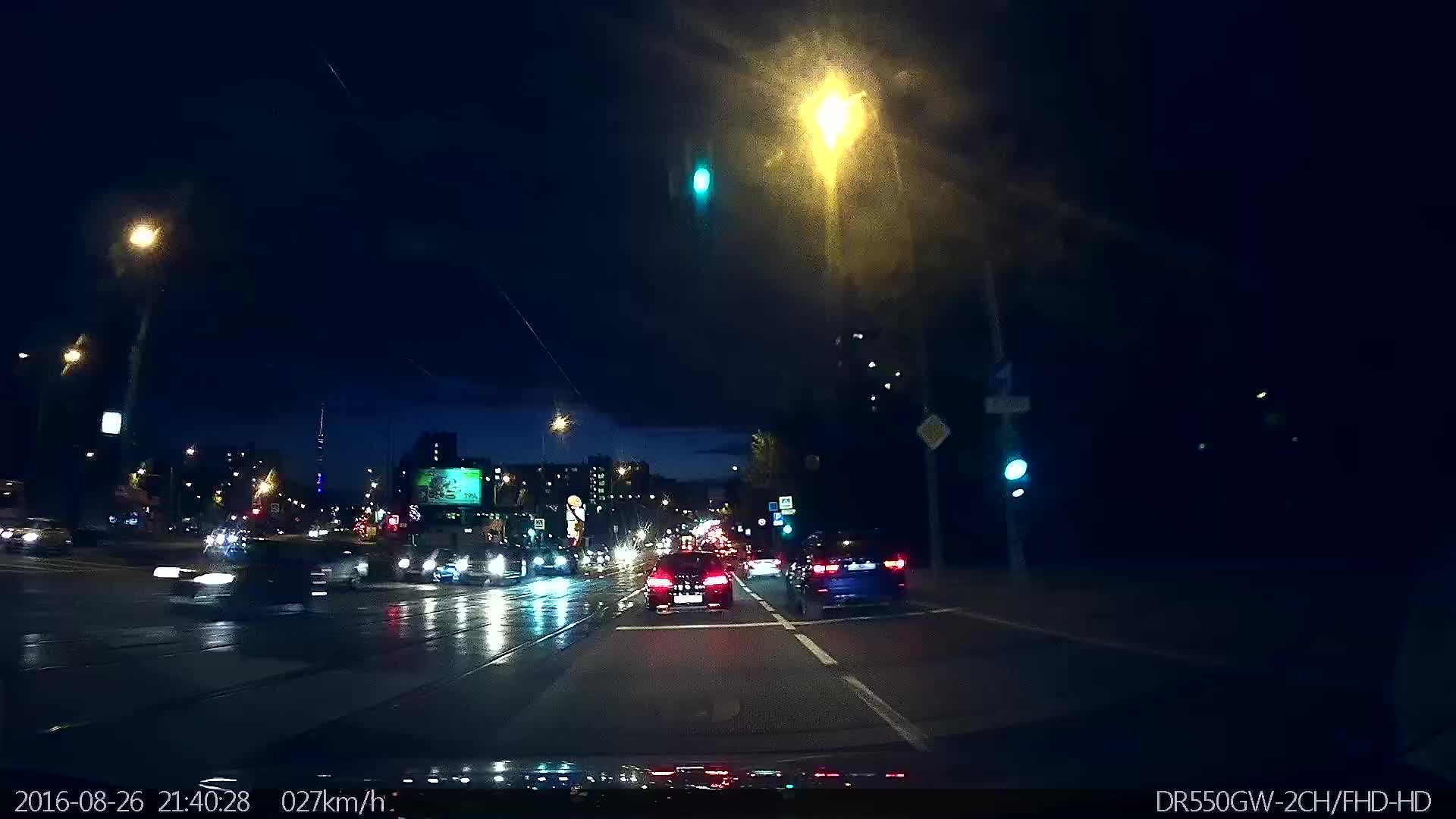This color photograph captures a vibrant street scene at night. At the bottom left of the image, partially legible text reads "2016/08/25" with additional notations, likely indicating time and speed, although somewhat difficult to decipher. On the right side, more text appears to read "DRSS 50GW" followed by a sequence of numbers ending in "HD."

In the foreground, the taillights of multiple cars are visible, illuminating the dark road ahead. A broken white line divides the lanes. Streetlights line the road, with one particularly prominent bright yellow lamp at the top of the image, casting a glowing aura that almost overwhelms the dark blue night sky. Adjacent to it on the left is a paler blue streetlight providing a softer illumination.

The left side of the road includes another lane where cars are heading towards the viewer. The headlights of these approaching cars create reflections on the slightly glistening road surface, adding to the contrast and depth of the scene. The interplay of lights and reflections creates a vivid and dynamic nighttime urban landscape.